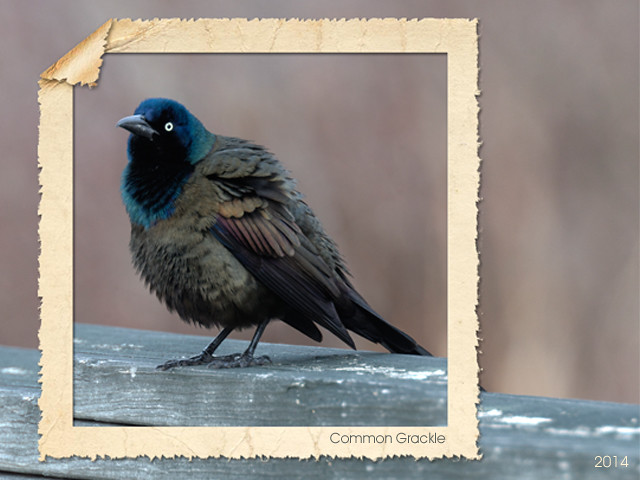This detailed photograph captures a Common Grackle in its natural habitat. The bird, primarily dark gray with a striking deep blue head and neck, stands perched on a blue-painted wooden railing, surveying its surroundings with its sharp, light blue beak and distinctive white and black eyes. The image employs a nature-documenting style, emphasizing the bird's features and species information. A photo-edited, torn-paper styled frame zooms in on the bird, and includes the Common Grackle's name in black font at the bottom right of the frame. The frame's top left corner folds slightly downward, adding a textured dimension to the presentation. The wooden railing beneath the bird serves as its perch, while a blurry, out-of-focus background of trees and leaves enriches the scene, ensuring the bird remains the focal point. In the very bottom right corner of the overall photograph, the year "2014" appears in white font, marking the time of the capture. The bird's rotund body showcases shades of blues, grays, and hints of greenish and reddish tones, making it a fine example of the species' vibrant plumage and robust form.